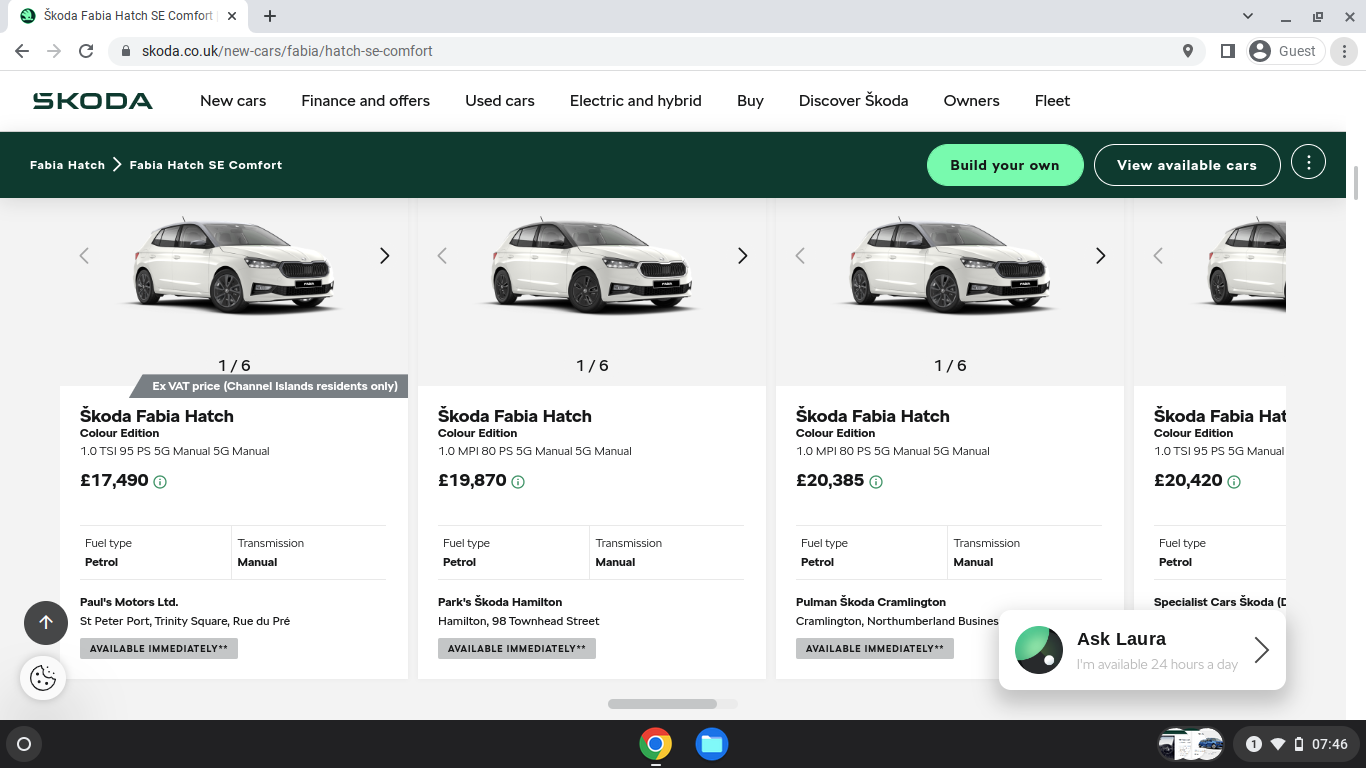The image shows a webpage from SCOTA's website, scota.co.uk/newcars/Fabia/hatch-SE-comfort. The screen displays multiple elements in black text, beginning with "SCOTA" at the top. Below, there is a navigation menu with links for "New Cars," "Finance & Offers," "Used Cars," "Electric & Hybrid," "Buy," "Discover SCOTA," "Owners," and "Fleet."

Following the top navigation, there is information about the SCOTA Fabia Hatch SE Comfort model. Two buttons are prominently featured: a green "Build Your Own" button and a "View Available Cars" button. Additionally, a circular icon with three dots is present, likely for more options.

Further down, there is a section labeled "SCOTA Fabia Hatch Color Selection," listing various models and their specifications:
1. A SCOTA Fabia Hatch priced at £17,490 with a petrol engine and manual transmission, available immediately at St. Peter's Park, Trinity Square, Roots of Pro.
2. Another SCOTA Fabia Hatch priced at £19,870, also available immediately.
3. A third SCOTA Fabia Hatch listed at £20,385, available immediately.
4. Lastly, a SCOTA Fabia Hatch Color Edition priced at £20,420.

Overall, the webpage provides detailed information on different SCOTA Fabia Hatch models, availability, and customization options.